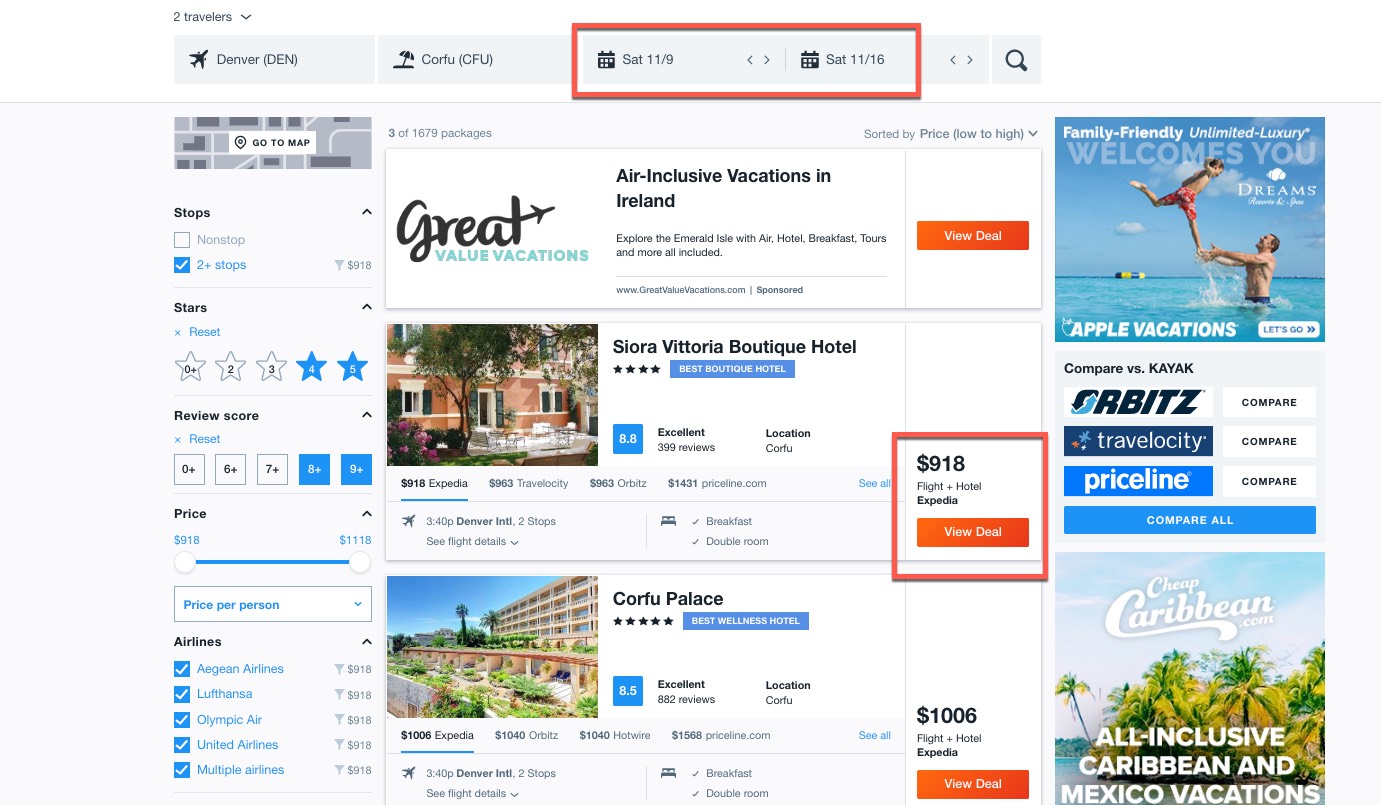**Detailed Descriptive Caption:**

This image is a screen capture from a travel booking website, likely showcasing flights and hotels for a specific trip. The header features a black navigation bar with the text "To travelers" and a dropdown menu. The travel route is displayed as "Denver (DEN)" accompanied by an airplane icon, and "Carrefour (CFU)" with an umbrella icon, indicating the destination. The travel dates are highlighted in orange, showing departure on Saturday, 11/9, and return on Saturday, 11/16, both marked with calendar icons. 

Below the header, there are several interface elements: gray arrows, a magnifying glass icon indicative of a search feature, and a 'Go to Map' button. A submenu in white lists various filters and sorting options. This includes a blue checkbox labeled "Two Stops," a star rating filter where four and five stars are selected in blue, and white stars for other ratings. A review score filter is set to show results rated between 8 and 9.

Price filters show a range from $916 to, presumably, $1,118, though the text is somewhat blurry. A blue box highlights the option to filter by "Price per Person." Additionally, several airlines are listed in blue, including Aegean Airlines, Lufthansa, Olympic Air, United, and a category for multiple airlines.

An advertisement on the right promotes "Great Value Vacations," specifically air-inclusive trips to Ireland, with an orange and white "View Deal" button. The ad further describes the package as including air travel, hotel stays, tours, and more, encouraging exploration of the Emerald Isle.

Further down, hotel listings are presented. The first is the "Sierra Futura Boutique Hotel," rated 8.8, with a price of $918 and an image showing an orange exterior of the building. Following this is the "Corfu Palace," priced at $1,006, rated 8.5, and also accompanied by an orange and white "View Deal" button.

Additional ads include one from "Apple Vacations," featuring a father throwing his child into the air while in the water, and buttons for comparing prices on different platforms like Kayak, Orbitz, Travelocity, and Priceline. There's also an ad promoting "Cheap Caribbean," focusing on all-inclusive vacations in the Caribbean and Mexico.

Overall, the screen capture provides a comprehensive snapshot of travel options, filters, and advertisements for vacation planning.